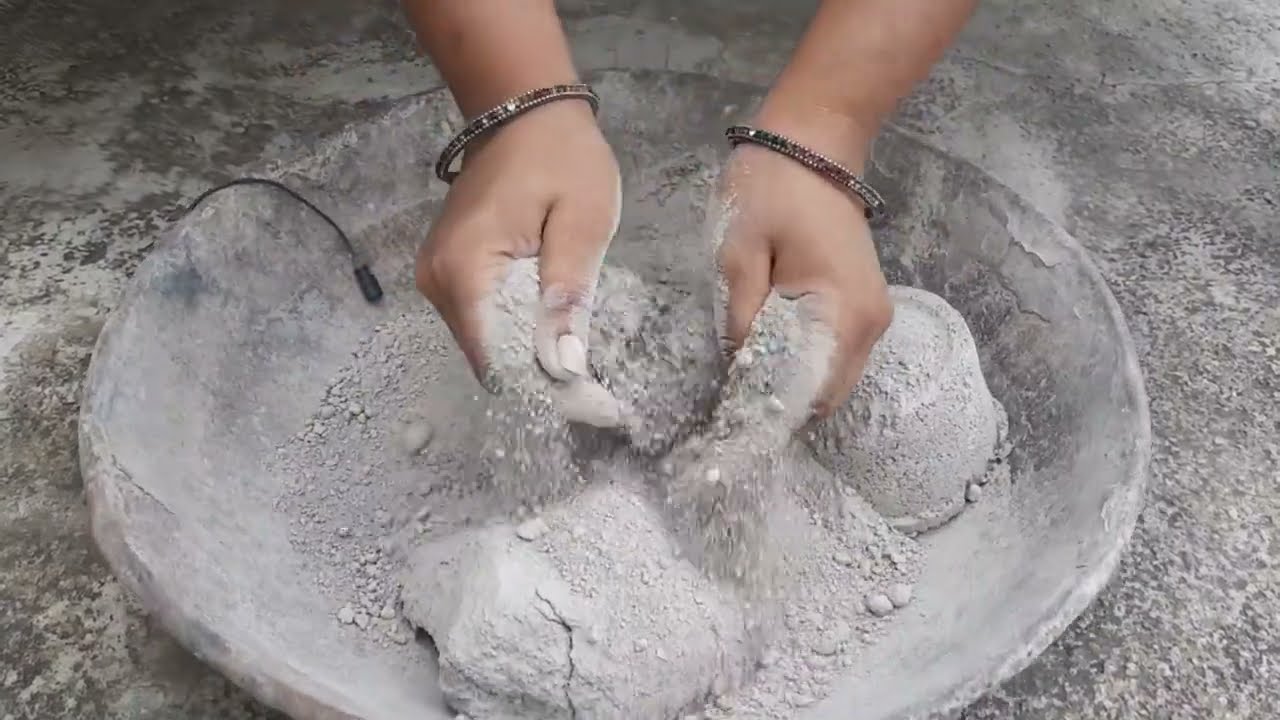The photograph captures a close-up view of a large, shallow stone bowl partially filled with gray, powdery dust that resembles ash, cement, or soil. The bowl is placed on a ground with mixed tones of white, gray, and black. Emerging from the top edge of the image are two brown hands, covered in and sifting through the gray dust, allowing it to flow through their fingers. Each wrist is adorned with thin, multicolored bracelets, contributing a subtle but noticeable detail. A thin black wire, possibly a microphone cord, drapes over the edge of the bowl, adding an element of curiosity to the scene. The setting is marked by a cohesive palette of gray hues, emphasizing the textural contrast between the hands, the dust, and the stone surface.